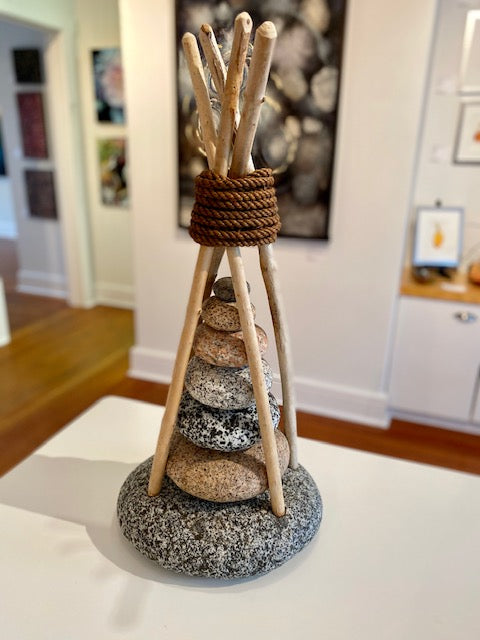The image features a decorative art piece positioned on a white countertop, likely in a kitchen or an open-layout house. The background is blurred but reveals wooden floors, white walls adorned with various pieces of art, and a white cabinet with a wooden top. The countertop hosts an intricate arrangement of smooth, tan sticks forming a tipi structure, held together by dark brown rope tied about an inch and a half to two inches from the top. Inside this tipi, a stack of six stones is carefully balanced from bottom to top. The stones, set on a slightly large circular stone base with black speckles, vary in color and texture. From bottom to top, the stones include a tan rock with brown speckles, a white rock with black speckles, a white rock with tan and black speckles, a reddish-brown rock, a light tan rock with dark brown speckles, and finally, a solid brown rock at the top. This harmonious blend of natural elements evokes a sense of zen and artistic symmetry.